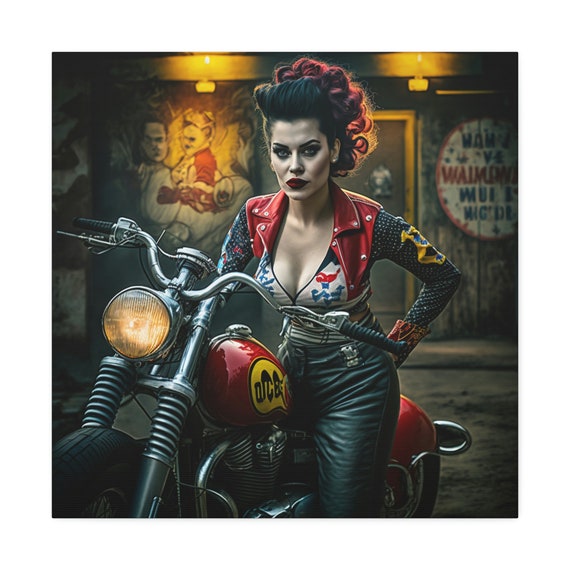A striking depiction of a woman seated on a shiny, new red motorcycle, illuminated by two yellow lights from a building behind her. The motorcycle features a prominent yellow decal with an indistinct, possibly dice-related, black text between the seat and handlebars. The woman sports a distinctive hairstyle: black hair with the front curled up and varying red and purple tints in the back, complementing her striking white makeup and black lipstick. She is dressed in a colorful, eclectic outfit comprising a red-collared jacket adorned with silver studs, black sleeves with white dots, and splashes of red, blue, and yellow, paired with sleek black leather pants. In the background, the slightly out-of-focus building shows some graffiti and a door trimmed in gold or yellow. Also visible is a sign on the right that is outlined in red, though the text remains unreadable. The image suggests an AI-generated origin due to inconsistencies, including the woman's mysteriously absent right arm.